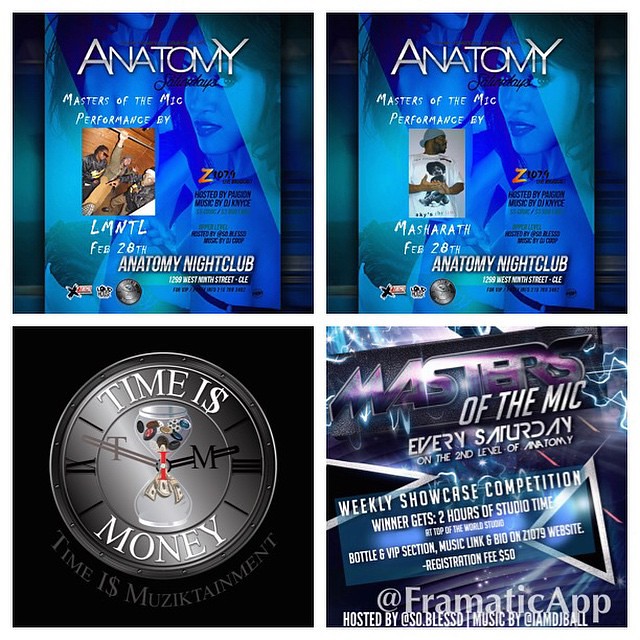The image is divided into four equal square pictures separated by white lines forming a cross. The top two pictures are promotional flyers for events at Anatomy nightclub, both featuring a blue and green background with a faded image of a woman. The top left flyer advertises a performance by LMNTL on February 28th and includes an image of three black men. The top right flyer, with the same background, advertises a performance by Masheroth, depicted as a single black man wearing a Biggie Smalls t-shirt and a gray beanie cap. Both flyers have “Anatomy Saturdays” prominently displayed.

In the bottom left quadrant, a close-up image of a clock is shown with the title “Time is Money,” where the 'S' is stylized as a dollar sign. The clock face features an hourglass filled with items reminiscent of poker chips. Below the clock, the text “time is musictainment” is visible.

The bottom right picture is another advertisement for the Anatomy nightclub, specifically for the “Masters of the Mic” event, held every Saturday on the second level. This flyer highlights the weekly showcase competition details, including a registration fee of $50, and promises rewards such as two hours of studio time, a bottle, a VIP section, and the music link on the Z1079 website.

Overall, the composite image dynamically captures the vibrancy and variety of events at Anatomy nightclub through detailed and engaging advertisements.